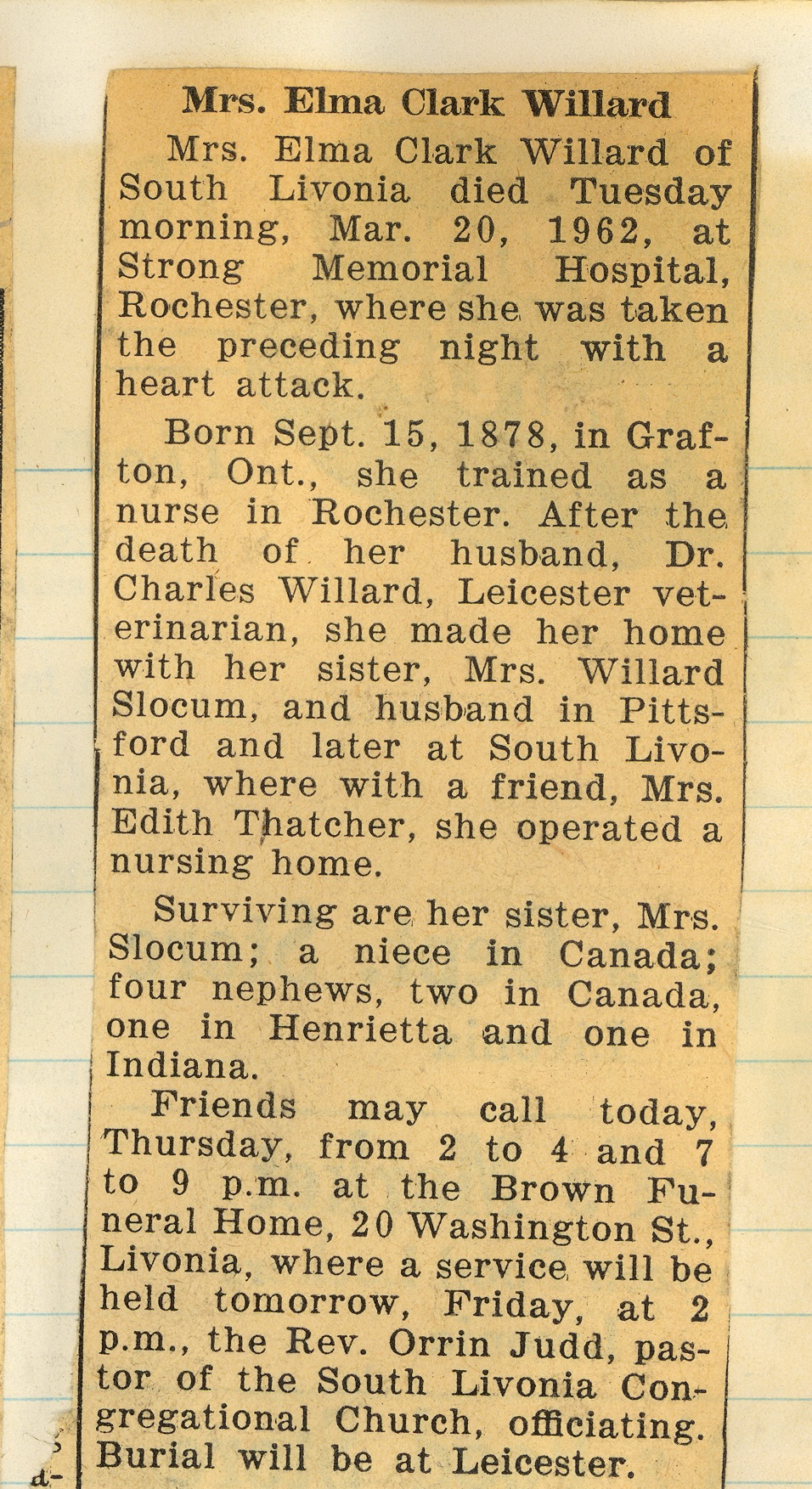The image showcases a centrally placed newspaper clipping set against the backdrop of yellow legal pad paper. The clipping, an aged and yellowed obituary, commemorates Mrs. Elma Clark Willard of South Livonia, who died on Tuesday morning, March 20th, 1962, at Strong Memorial Hospital in Rochester following a heart attack. Born on September 15th, 1878, in Grafton, Ontario, Mrs. Willard trained as a nurse in Rochester. After the death of her husband, Dr. Charles Willard, a Leicester veterinarian, she lived with her sister, Mrs. Willard Slocum, in Pittsburgh, and later in South Livonia, where she co-operated a nursing home with a friend, Mrs. Edith Thatcher. She is survived by her sister, a niece in Canada, and four nephews—two in Canada, one in Henrietta, and one in Indiana. Friends were invited to call on Thursday from 2 to 4 p.m. and 7 to 9 p.m. at the Brown Funeral Home, 20 Washington Street, Livonia, with a service to be held on Friday at 2 p.m. officiated by Reverend Orrin Judge, pastor of the South Livonia Congregational Church. Burial followed at Leicester. The obituary is printed in black font on the roughly cut newspaper snippet, which is the focal point of the image. The colors visible include white, yellow, black, and light blue, accentuating the worn texture and somber tone of the historical document.